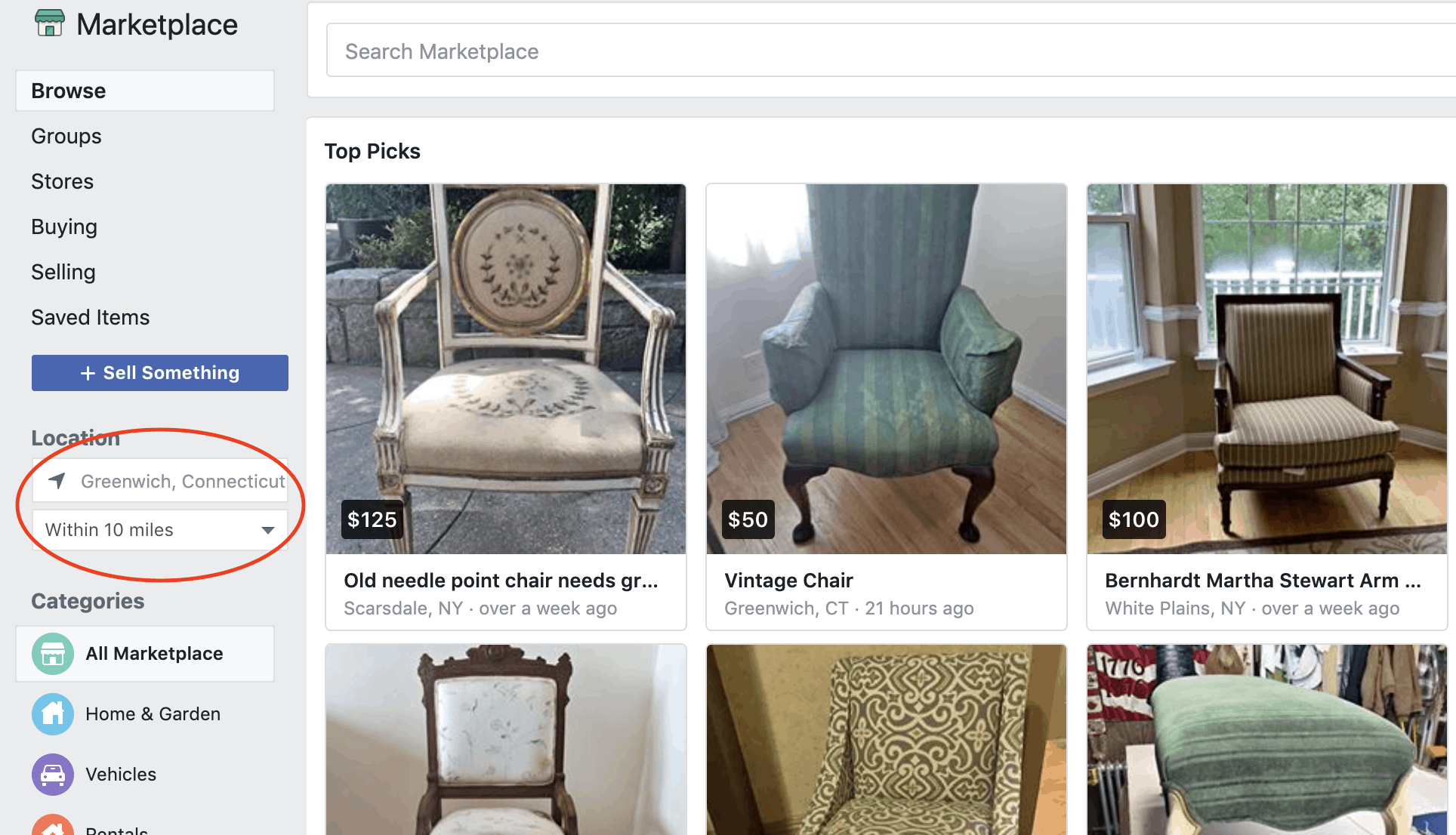This is a detailed screenshot from a marketplace platform, possibly Facebook Marketplace. On the far left side of the image, a vertical light grey banner occupies nearly a quarter of the frame. At the top of this banner is a small, cartoonish image of a house with white walls, a blue roof, and a blue door. Next to the house icon, "Marketplace" is written in black text. Below this, the options available are "Browse," "Groups," "Stores," "Buying," "Selling," and "Saved Items." There is also a blue tab labeled "Sell something" in white text. Beneath this, it states the location as "Greenwich, Connecticut," with an option for "Within 10 miles" highlighted in a red oval. The "Categories" listed include "All Marketplace," "Home and Garden," "Vehicles," and partially visible, "Rentals."

To the right, a section titled "Furniture. Top Picks" displays various items. Among them is an old needlepoint chair priced at $125. Another item is a vintage chair featuring light and dark blue stripes with wooden legs, priced at $50. A Bernat Martha Stewart armchair with dark wood and white and olive green striped upholstery is listed for $100. The bottom left shows a chair upholstered in velvety white material with a dark brown wooden frame. Another chair features an olive green and cream pattern reminiscent of certain carpet and drapery designs. Finally, there is a small, backless chair that resembles a footstool, with light greenish-blue striped upholstery and white legs.